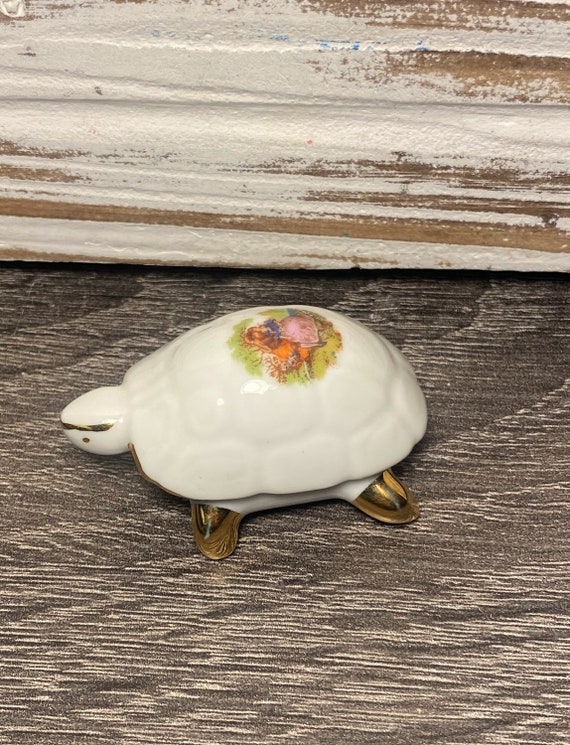The image features a porcelain turtle figurine adorned with gold feet, resting on a brown carpet with white streaks. The turtle itself is primarily white, with a detailed and colorful pattern on its shell. The intricate design on the shell depicts a nature scene with a male and female couple. The female, dressed in a pink dress, is accompanied by a figure in an orange outfit, both set against a backdrop of lush green fields. Additional elements in the illustration include a basket filled with flowers and a tree in the background. The turtle's head is oriented towards the left, marked by a simplistic black line for a mouth and a discreet dot beneath it. The figurine is positioned in front of a partially painted wall, blending hues of white and brown, and is adjacent to the base of a white and brown coffee table.